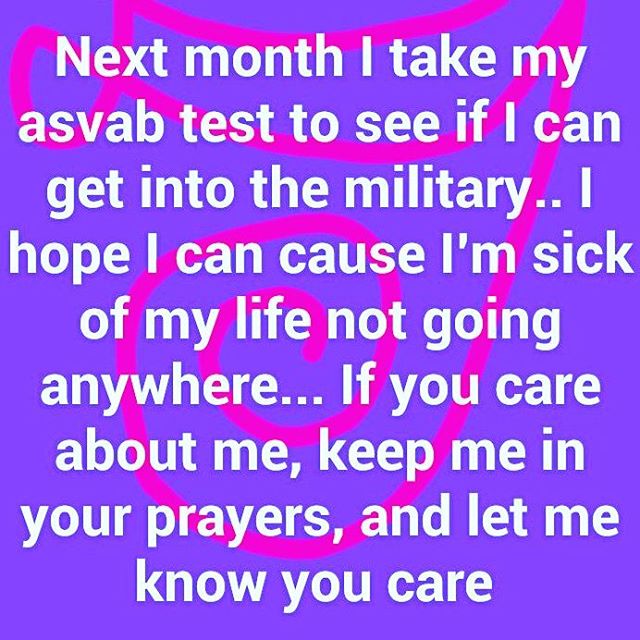This image displays a rectangular, horizontal graphic with a purple background and a notable pink swirl reminiscent of a magic marker tracing across the page. Dominating the visual is white text that conveys a heartfelt message: "Next month, I take my ASVAB test to see if I can get into the military. I hope I can because I'm sick of my life not going anywhere. If you care about me, keep me in your prayers and let me know you care." The overall composition suggests an earnest plea for emotional support, possibly intended for social media, against a simple yet vibrant setting of purple, pink, and white.